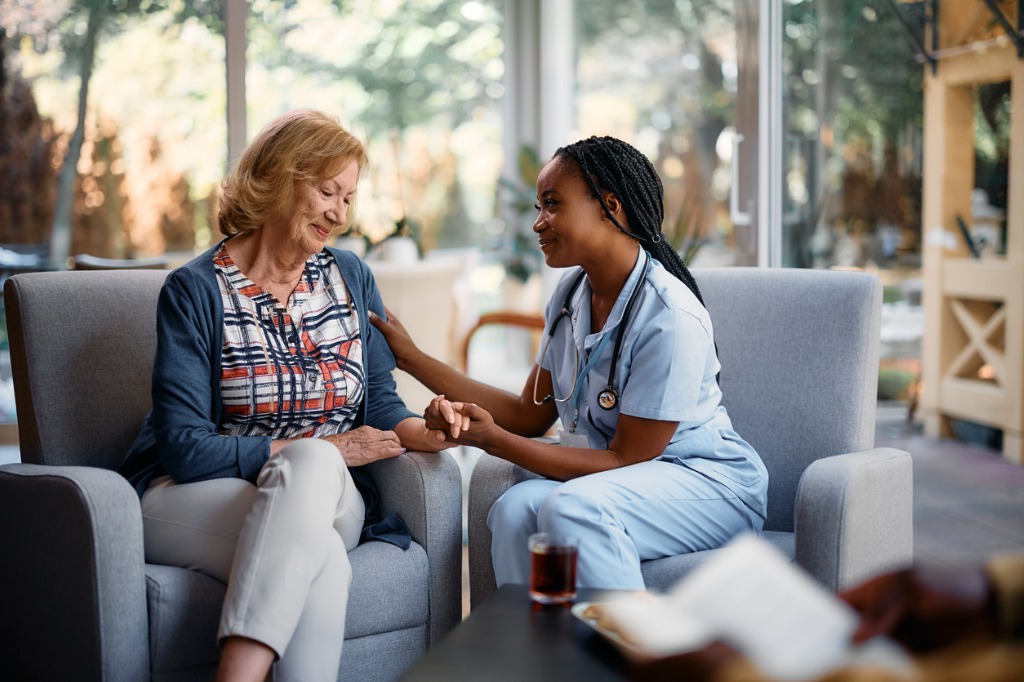In a cozy, well-lit interior setting with large windows offering a blurry view of trees and the sky outside, an older white woman and a younger African-American nurse are seated in cushioned gray chairs. The older woman, with medium-length reddish-blonde hair, is dressed in white capris, a blue, white, and red plaid shirt, and a cardigan. The nurse, sporting thick braids pulled back into a ponytail, is wearing blue scrubs and a stethoscope around her neck. They are engaged in a warm interaction, the nurse gently clasping the older woman's hand while placing her other hand on her arm. On the table in front of them sits a dark-colored drink and some snacks, adding a homey feel to the environment, which could be a senior home or a hospital recreation area. The overall atmosphere is serene and comforting, with natural light flooding the space through the expansive windows.